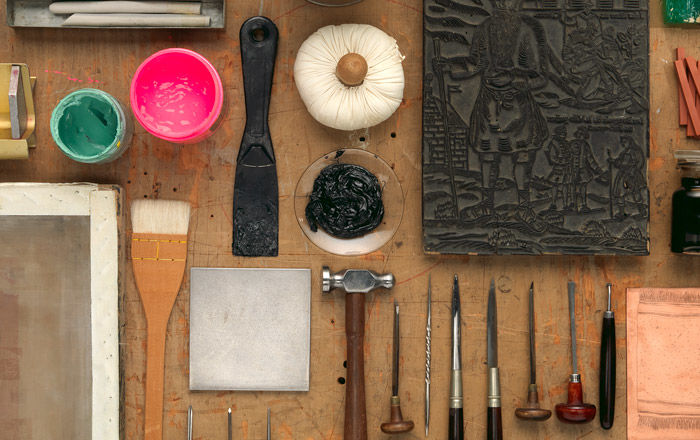This photograph captures an exceptionally neat and well-organized workshop, primarily focused on a plywood-covered wall arranged with various tools. Prominent tools include awls, hammers with dark brown handles, screwdrivers, and knives, all hung in an orderly manner. The plywood displays an assortment of items, such as a ball of white string hanging from a knob, three jars that appear to contain grease or lubricant, and small bowls with nails. Visible on the plywood are intricate lithographs and a decorative plaque, one potentially depicting scenes of ancient people, adding a touch of art to the workspace.

Central to the image is a well-worn, light-brown workbench, marked with paint and other signs of use, adding character to the scene. On the bench, there is a variety of tools and materials: a black paint spatula, a white-and-brown paintbrush, jars of pink and lime green paint, and a white tray containing black paint. The setup also includes a slightly cropped wooden frame on the left and a pink canvas to the bottom right. The meticulous arrangement of over a dozen different tools and supplies suggests a workspace where creativity meets meticulous organization.